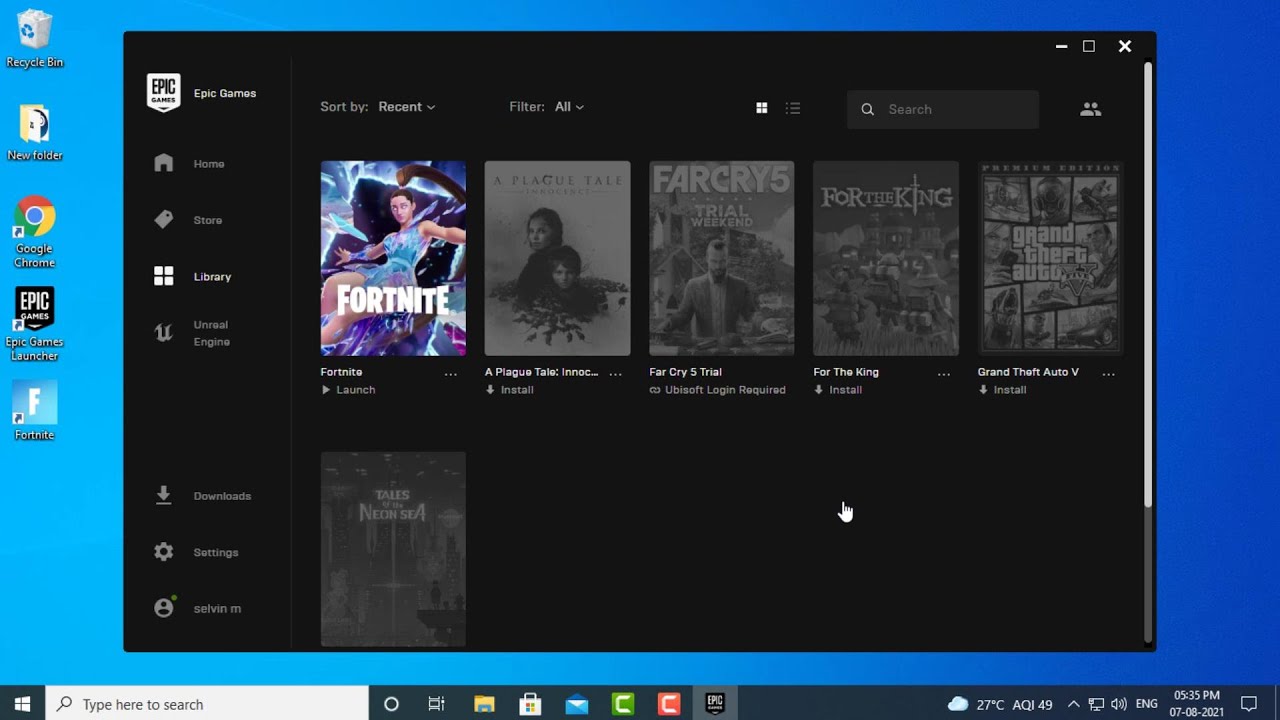The image depicts a horizontally rectangular screenshot of a computer monitor displaying a user's desktop. The background gradients from light blue on the left to darker blue on the right. Notably, the left side of the screen features several desktop icons arranged vertically, starting with the Recycle Bin at the top, followed by a New Folder, Google Chrome, Epic Games Launcher, and Fortnite icons.

Along the bottom of the screen, the Windows toolbar is visible, showing the Windows icon on the left, followed by a search field, a File icon, a Store icon, and a Mail icon. On the far right of the toolbar, the date and time are displayed as 5:35 PM, July 8, 2021.

The remainder of the screen is dominated by an open application, the Epic Games Launcher, which has a black background. At the top of the launcher interface, sorting options are available, with 'Sort by' followed by a selected drop-down menu labeled 'Recent.' Additionally, there is a 'Filter by' drop-down set to 'All' and a search field to the right.

Beneath these filters, a row of five game icons is displayed. Four of them, located from the second to the fifth positions, are grayed out, while the first game on the left, Fortnite, is displayed in full color, indicating it is likely selected or available for interaction.